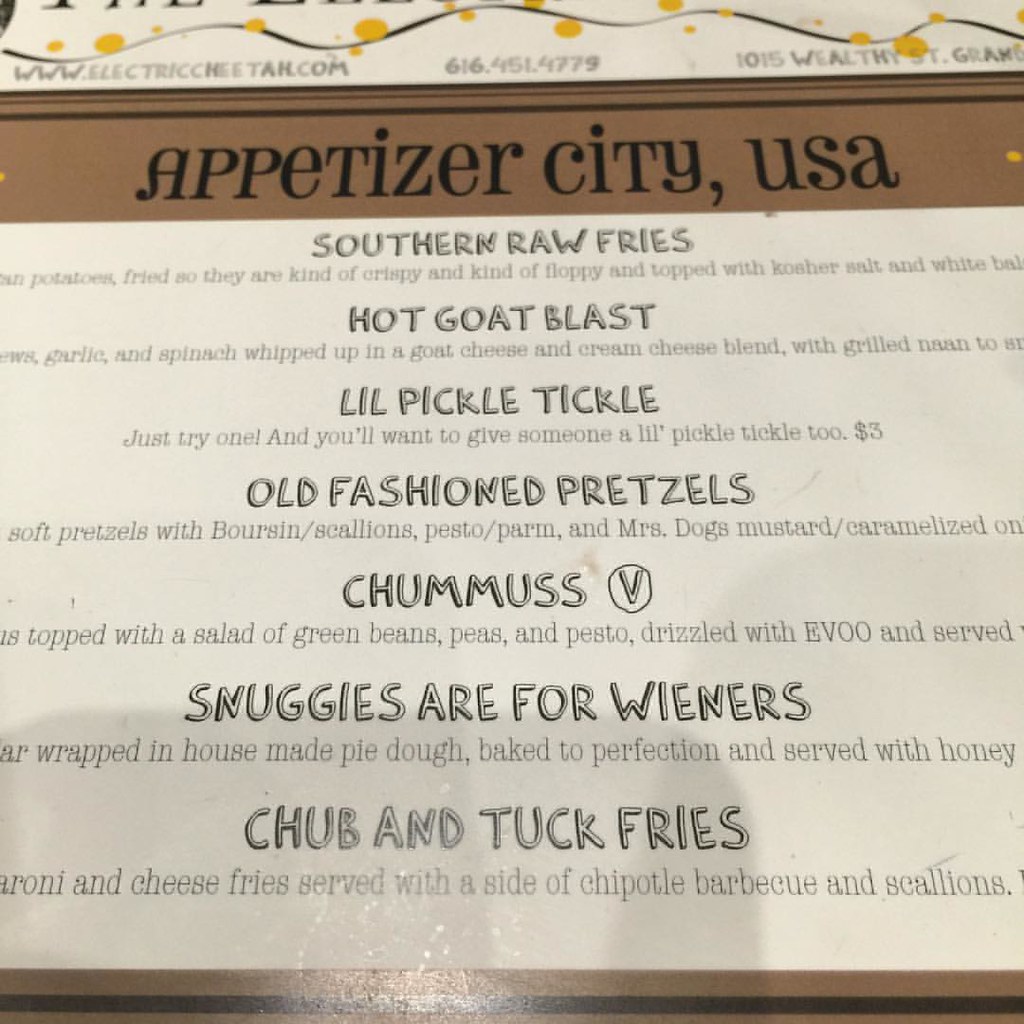This image features a menu from a place called "Appetizer City USA." The poster is a light tan color, though its very top section is cut off. Displayed at the top is a dark brown rectangle with "Appetizer City USA" printed on it. Above this rectangle, a website is listed: electriccheetah.com, along with the phone number 616-451-4779 and the address 1015 Wealthy Street, G-R-A-M. Above these details is a decorative swoopy line accented with small yellow dots.

Underneath the "Appetizer City USA" title, the menu lists the following specials:

1. **Southern Raw Fries** - Potatoes fried to a texture that is both crispy and floppy, topped with kosher salt and an incomplete description ending with "white B-A-L."
   
2. **Hot Goat Blast** - A blend of garlic and spinach whipped into goat cheese and cream cheese, served with grilled naan. The rest of the description is cut off.

3. **Little Pickle Tickle** - Encourages you to try one, promising that doing so will make you want to give someone a "Little Pickle Tickle" too.

4. **Veedahollers Old Fashioned Pretzels** - Soft pretzels served with boursin cheese, scallions, pesto, parmesan, and Mrs. Dog's mustard. Partially visible text hints at caramelized onions.

5. **Chummas (V)** - A dish topped with a salad of green beans, peas, and pesto, drizzled with extra virgin olive oil (EVOO). The rest of the description is cut off.

6. **Snuggies are for Wieners** - Incomplete description; it mentions being wrapped in house-made pie dough, baked to perfection, and served with honey.

7. **Chubb and Tuck Fries** - Described as fries served with chipotle barbecue and scallions. The mention of "macaroni and cheese" is partially cut off.

The menu's layout suggests that it is either laying on a table or displayed on a wall, with each food item title capitalized and followed by descriptive text.